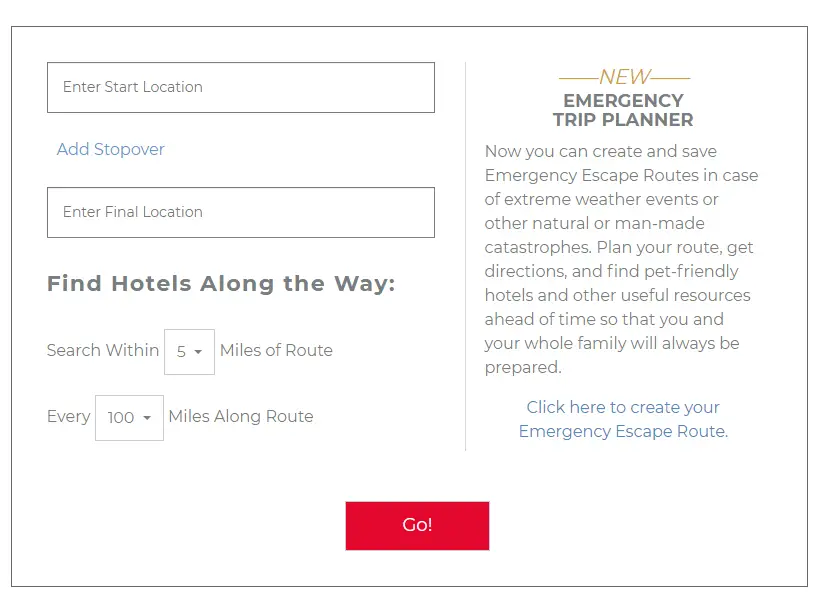The image depicts an interface designed for planning emergency escape routes. It features multiple fields for user inputs, including "Enter start location," "Add stopover," and "Enter final location." Adjacent to these fields, there is a prompt encouraging users to "Find hotels along the way," with additional options to "Search within 5 miles of routes" and "Every 100 miles along routes." A prominent "Go" button, highlighted in red, is situated below these input sections. 

To the right of these input fields, there is descriptive text introducing the "New Emergency Trip Planner." This tool enables users to create and save emergency escape routes in situations such as extreme weather events or other natural or man-made disasters. It offers features for planning routes, obtaining directions, and identifying pet-friendly hotels and other essential amenities ahead of time, ensuring comprehensive preparedness for all family members. 

The color scheme of the image consists of a white background with black text, and the "Go" button in red stands out for emphasis. A call-to-action at the bottom invites users to "Click here to create your emergency escape routes."